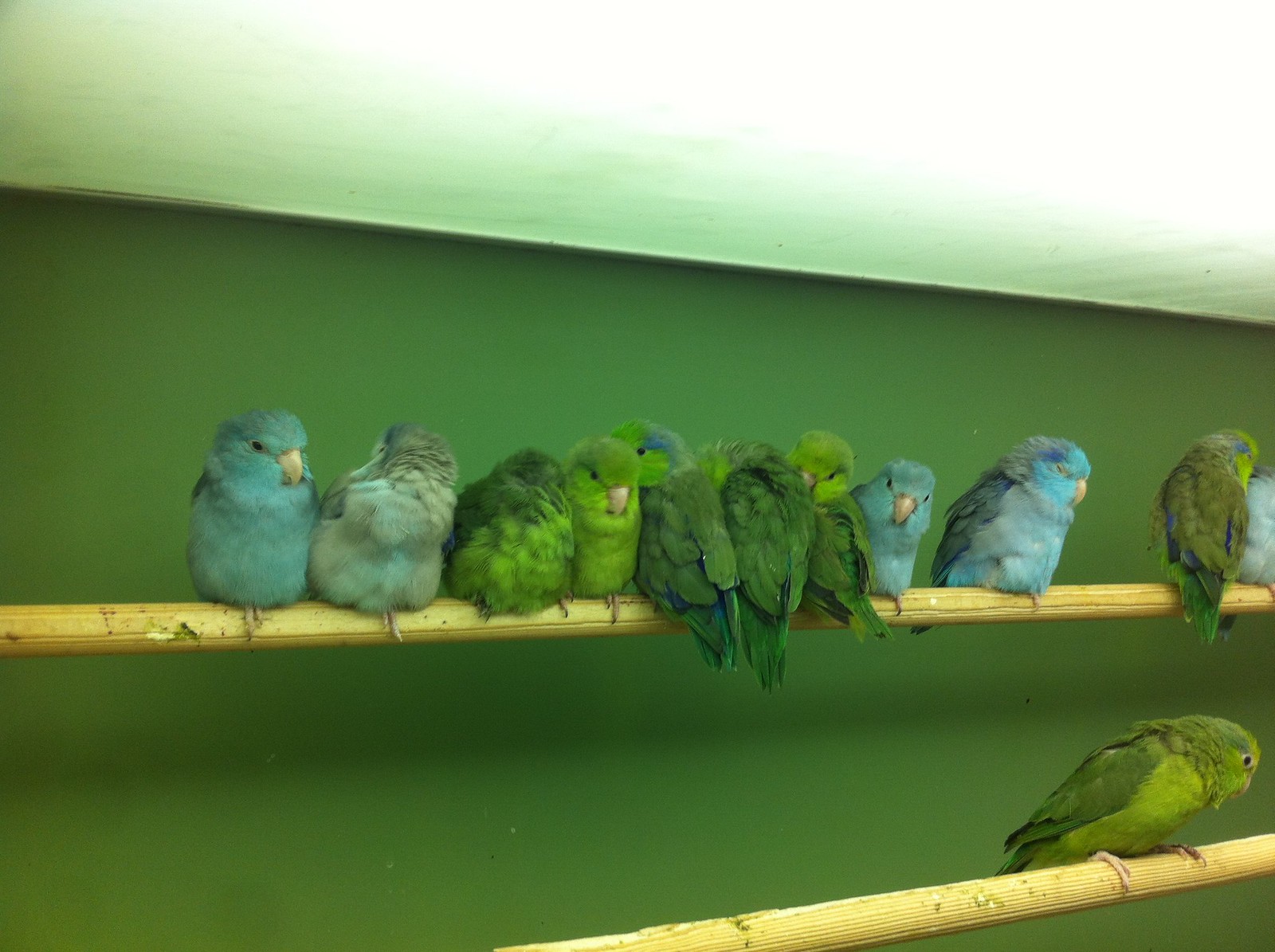The image depicts a group of small birds, possibly parakeets or lovebirds, perched against a green background wall with a white ceiling above. Two wooden roosting poles run horizontally across the image. The top pole is crowded with birds of varying colors, predominantly green and light blue, with some individuals exhibiting a mix of green, blue, and yellow. These birds are positioned side by side, with some facing forward and others turned towards the wall. The bottom pole features a single green bird perched by itself. The spacing between the birds on the top pole varies, with some perched closely together and others more spread out.